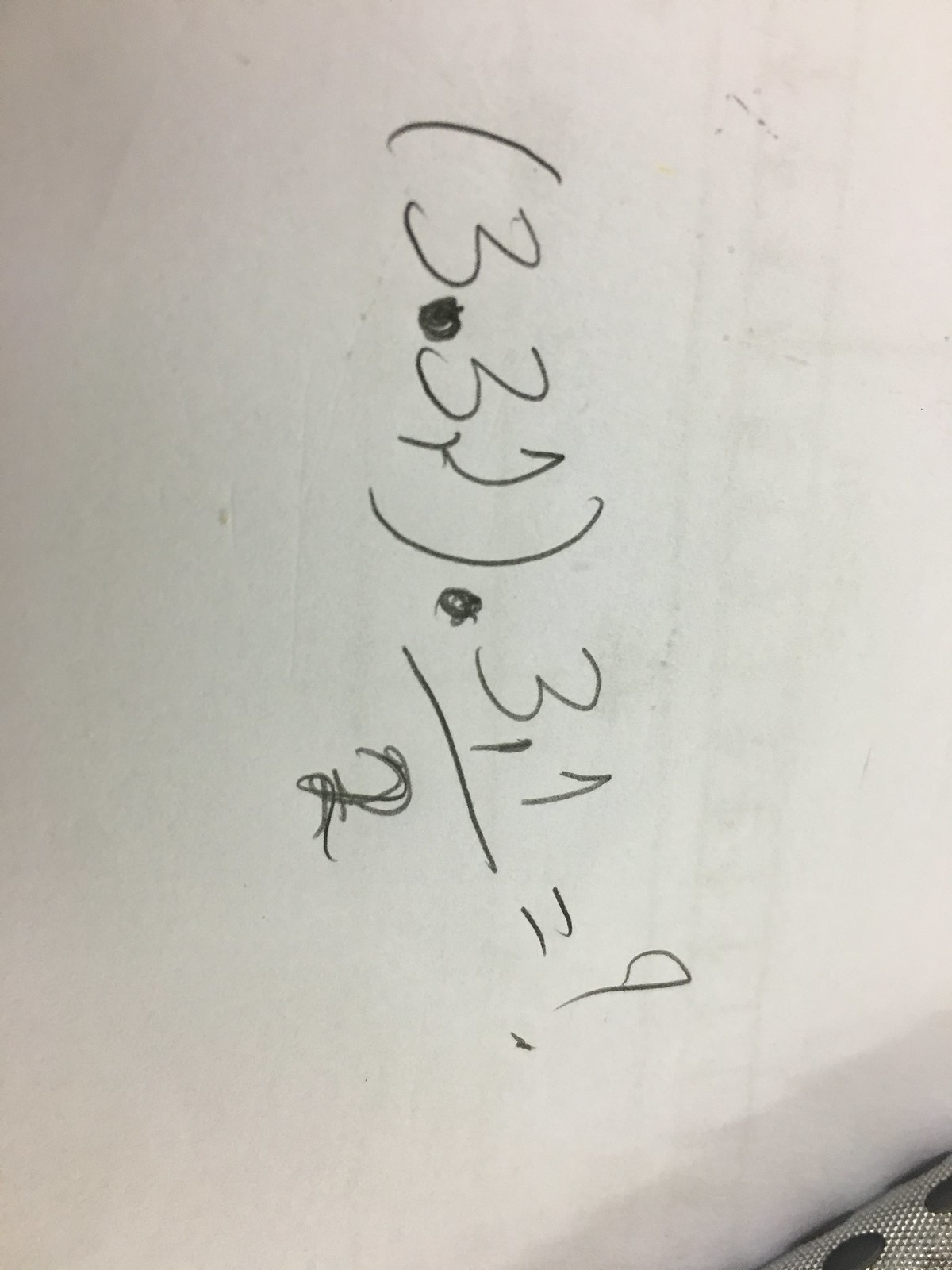This photograph, slightly tilted, showcases a handwritten mathematical formula on a white sheet of paper, using black pen ink. There are noticeable gray shadows cast across the paper. In the corner of the image, a partially visible white object with black circles can be seen, though it is not clear what the object is due to its limited visibility.

The formula on the paper is structured as follows: within parentheses, the numbers "3.3" are written, followed by another set of parentheses containing a somewhat illegible number that could be a "2." Adjacent to this, a dot is followed by the numbers "3" and "1." Below these, a line is drawn with a slightly messy "2" written beneath it. Finally, the equation ends with an equals sign and a question mark. The entire expression reads: (3.3 (indecipherable number)) · 3 1 / 2 = ?.